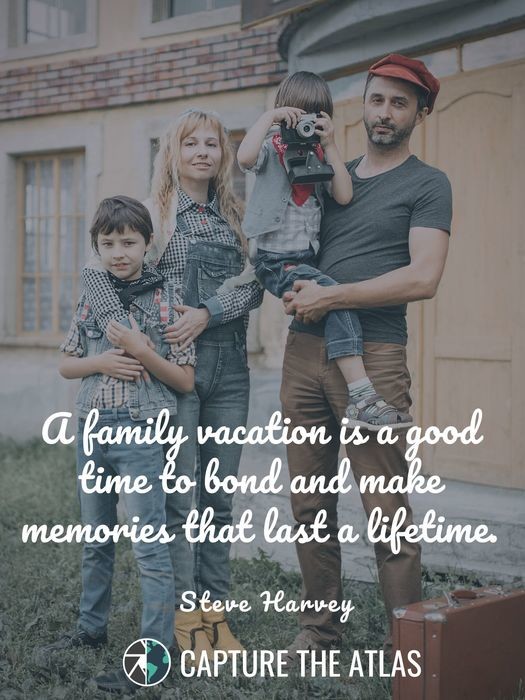The image portrays a family of four standing in front of a yellow building with white trim and brickwork accents. The father, positioned on the right, is wearing a red French-style beret, a gray cotton t-shirt, brownish jeans, and brown shoes. He is holding a young child who is lifting an instant camera, obscuring their face. To the left of the father is the mother, a blonde woman dressed in jean overalls with a checkered print undershirt and yellow-orange heeled boots. She has her arm around another child, who appears to be about 9 or 10 years old. This child is wearing a jean vest and jean pants, matching the mother's outfit theme. The family stands in front of yellow doors elevated by one or two white steps, and a suitcase is visible at the bottom right corner of the image. Superimposed text in white, handwritten-style digital font at the bottom of the photograph reads: "A family vacation is a good time to bond and make memories that last a lifetime." This quote is attributed to Steve Harvey, followed by a globe logo and the phrase "Capture the Atlas."